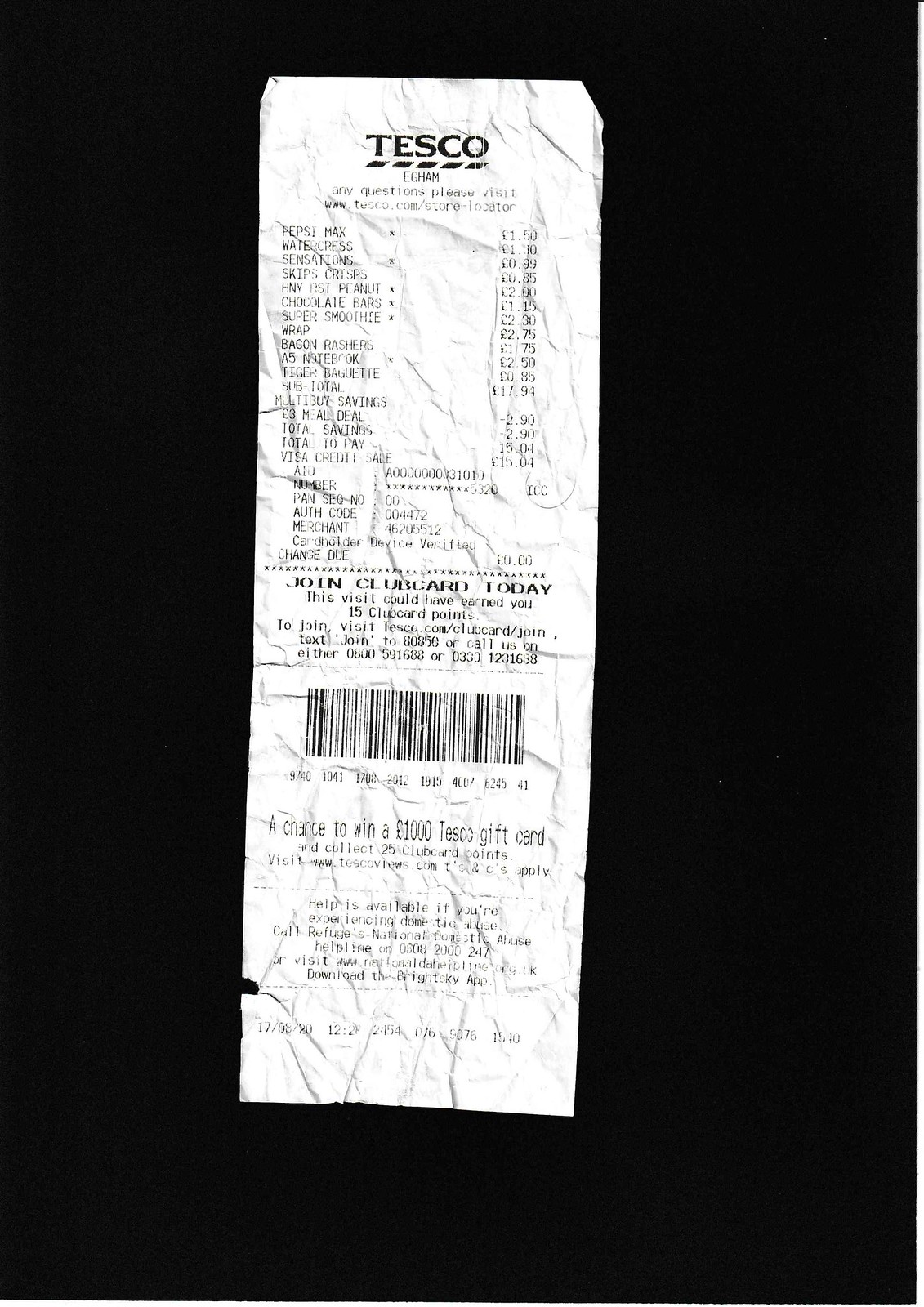In this black and white photo, the focus is on a vertically placed, heavily crumpled Tesco receipt, set against a pitch-black background. The receipt appears to have been scanned despite its significantly wrinkled and slightly torn condition at the lower left-hand corner. At the top, "Tesco" is prominently displayed in black letters, followed by a series of small, barely legible text detailing purchased items and their prices due to the crumpled state. Items such as Pepsi Max (£1.50), Watercress Sensations (£0.99), Skips Crisps (£0.85), peanuts (£2.00), chocolate bars (£1.15), a super smoothie (£2.30), a wrap (£2.75), bacon rashers (£1.75), an A5 notebook (£2.50), and a tiger baguette (£0.85) totalled to a subtotal of £17.94. Beneath the itemized list, the receipt mentions multi-buy savings and the prompt, "Join Clubcard today," suggesting opportunities to earn Clubcard points. The barcode and further text below offer a chance to win a £1,000 Tesco gift card and the potential to collect more Clubcard points. There are some numbers resembling a date and time, but they are too small to decipher.